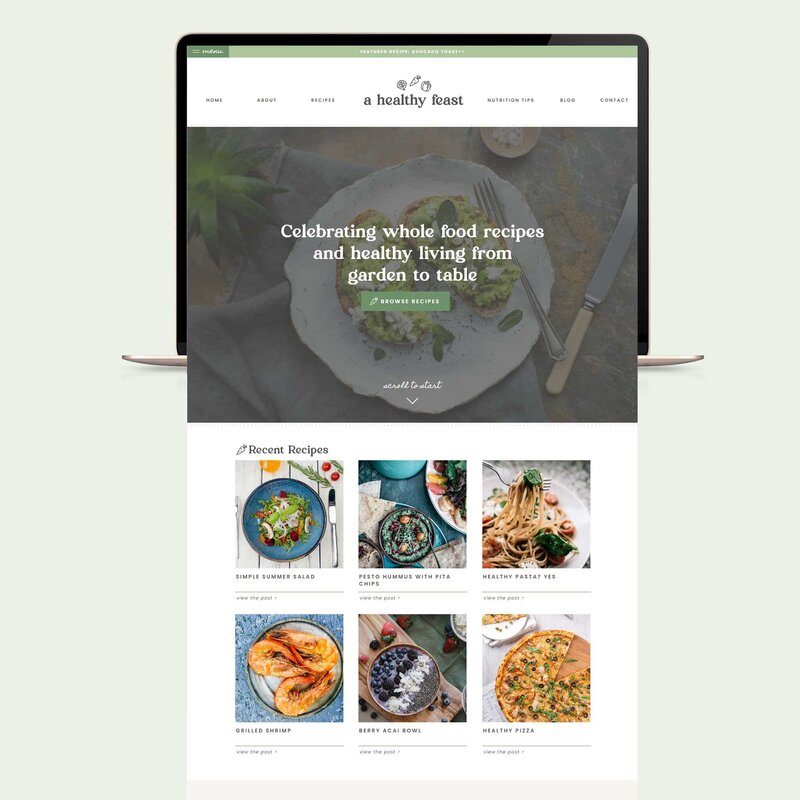Set against a clean, light gray background, this screenshot captures the detailed view of a computer monitor displaying an extended website interface. Behind this main monitor, the silhouette of a black computer screen is faintly visible. The website interface opens with a light gray header, followed by a white banner. Displayed in dark gray text from left to right, the menu options are: Home, About, Recipes, Nutrition Tips, and Contact.

Centered prominently in bold text, the website title reads "A Healthy Feast." Located above the title, there are three icons: a carrot on the left, a leaf in the center, and an apple on the right.

Directly below the title, the background showcases a slightly grayed-out image featuring a white plate with two pieces of what appear to be chicken breast. A silver fork is positioned to the right of the plate, accompanied by a knife. In the upper left corner of this image, there is a partial view of a plant. Overlaying this image in bold white text is the phrase "Celebrating Whole Food Recipes and Healthy Living from Garden to Table."